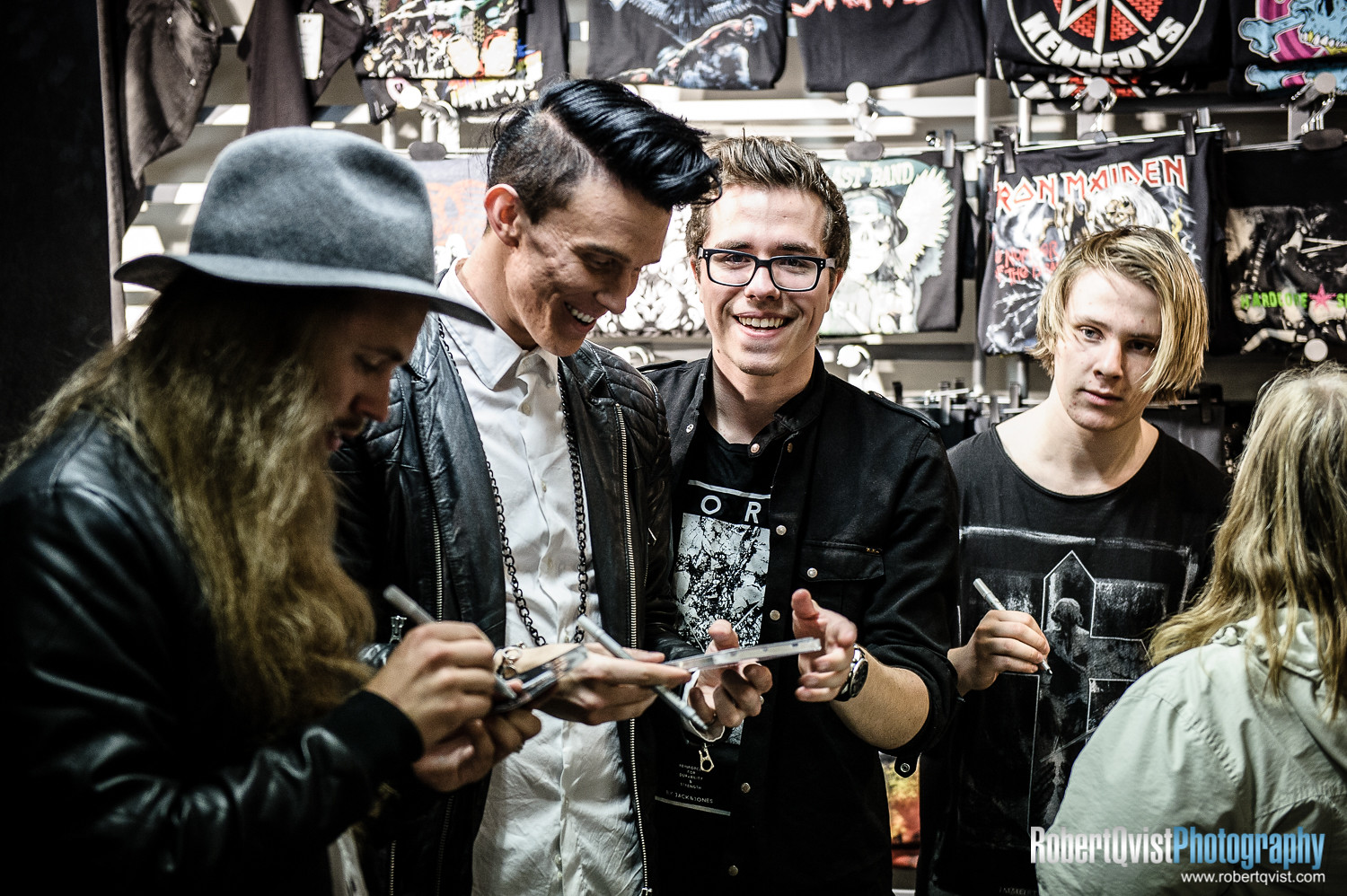In the image, we observe an autograph signing session likely set in a shop or market area, surrounded by rock and roll memorabilia. Four younger men are the focal point, preparing to sign autographs. The first man on the left dons a black jacket and glasses; the second, who is somewhat younger, sports long, blonde hair partially covering his face. The third man has short, black hair on the sides, longer on top, and wears a white shirt under a black leather jacket with a pendant. The last man, wearing a wide-brimmed black hat over his long, brown hair, also has a black leather jacket.

They are standing in a line from left to right: the first two hold cards and pens in their hands, presumably about to sign autographs. The two on the right face the camera directly, while the left two are slightly angled. T-shirts featuring bands like Iron Maiden and advertisements for Kennedy’s hang in the background, contributing to the rock and roll ambiance.

Additionally, we see part of another individual in the bottom right, only identifiable by a partial view of their jacket and the back of their head. A woman stands to the far right, likely waiting for an autograph. The image is credited to Robert Q Visit Photography, as indicated in the bottom right corner along with the website www.robertqvisit.com. The fans and signers alike are in high spirits, smiling warmly amidst the scene filled with memorabilia in various shades, including black, white, blue, and lime green.